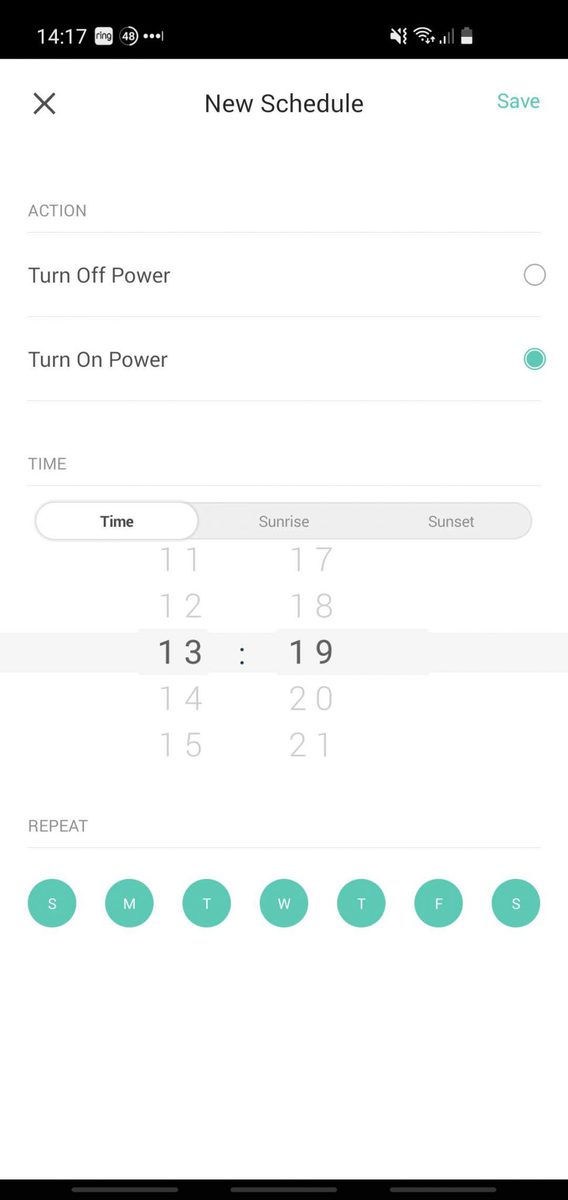Screenshot of a mobile device displaying a scheduling interface:

At the top of the phone screen, there's a black border showing the current time as 14:17 in the left corner, along with icons for Wi-Fi connectivity and a partially charged battery on the right. Below this, on a white background, there is a small 'X' in the upper-left corner, labeled "New Schedule" in the center, and a teal "Save" option to the right.

Further down, a heading labeled "Action" appears, accompanied by two selectable options: "Turn off power" and "Turn on power." The "Turn on power" option has been selected, indicated by a teal-colored circle next to it.

Below this, a "Time" heading is visible, with a clock interface set to 13:19. Underneath is another heading labeled "Repeat," displaying seven teal circles that represent the days of the week, marked with the abbreviations SMTWTFS.

The lower portion of the screen is plain white with no additional content, and the very bottom of the screen features a black band.